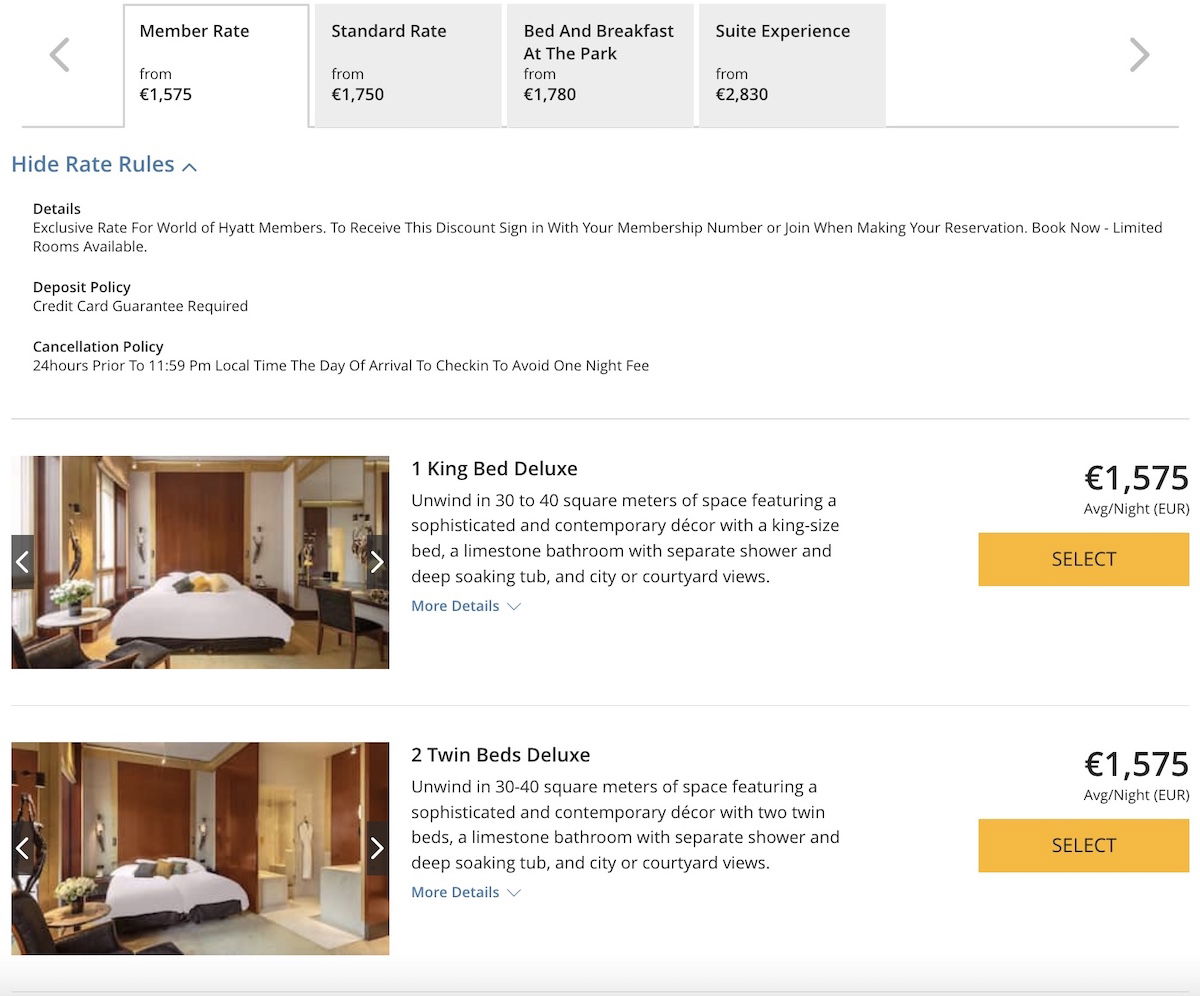In this image, a hotel booking website is displayed, showcasing various room options and rates. At the top of the page, the available rates for different membership statuses are listed as follows: Member Rate from $1575, Standard Rate from $1750, Bed and Breakfast at the Park from $1780, and Suite Experience from $2830. Below these rates, there is a notice explaining that World of Hyatt members can access exclusive discounts by signing in with their membership number or joining during the reservation process. The site encourages immediate booking due to limited room availability.

Further down, the website details the deposit policy, requiring a credit card guarantee. Additionally, the cancellation policy stipulates that guests must cancel 24 hours prior to 11:59 p.m. local time on the day of arrival to avoid a fee equivalent to one night's stay. 

The page also features examples of available rooms. The first example is a photo of a hotel room labeled "One King Bed Deluxe," which offers 30 to 40 square meters of space with sophisticated and contemporary decor. The second example is labeled "Two Twin Beds Deluxe," providing similar luxury and comfort with two separate twin beds.